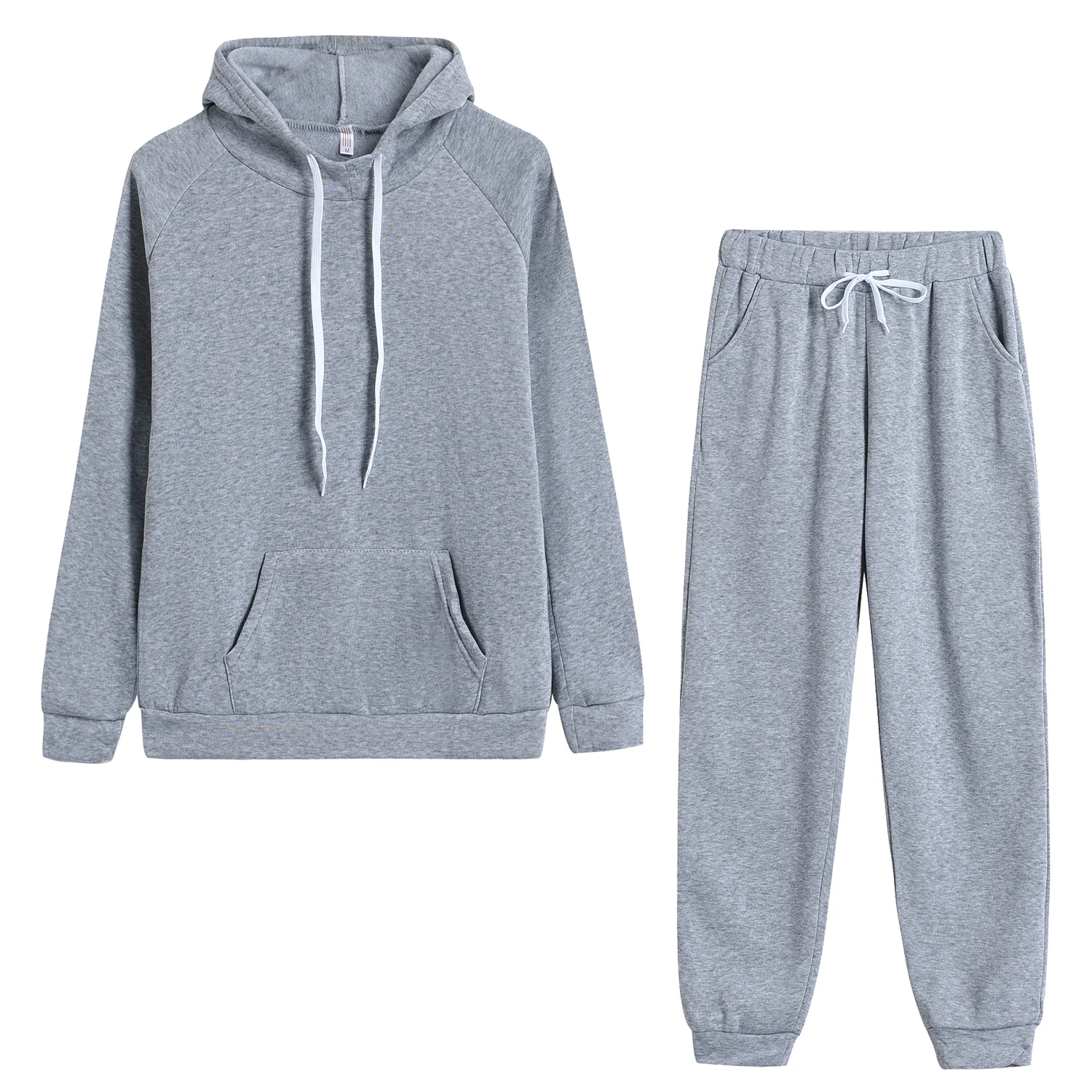The image displays a matching gray hooded sweater and sweatpants set against a solid white background. The gray color of both pieces is a heathered or sport gray. In the top-left corner, the hooded sweater features white drawstrings, a front pocket, and borders of consistent width at the wrists and hem. The sweatpants, positioned more towards the bottom-right of the image, also showcase a matching cuffed ankle and ruched waistband with a white drawstring for adjustable fit. The top of the sweatpants extends just below the shoulder level of the sweatshirt. Both pieces are coordinated in style, with the sweatpants featuring pockets on either side, and a tiny skinny tag visible inside the neck of the hoodie. The hood of the sweater is shown slightly squished, not fully extended. Overall, the outfit forms a cohesive and casual set with practical details suitable for sporty or relaxed activities.